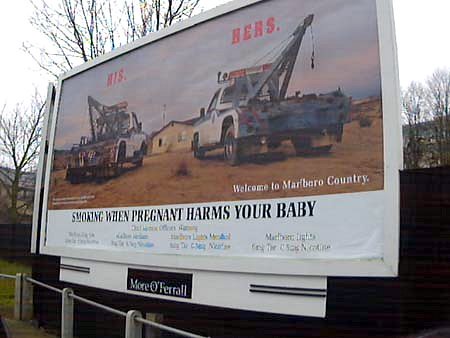The photograph captures a billboard situated outdoors, framed by a clear, gray sky and leafless trees, suggesting it was taken during the colder months. The billboard prominently features two tow trucks positioned against a desert-like background, facing each other. Red text labels the trucks as "his" on the left and "hers" on the right. Between them, a small house is distinguishable. In the lower right corner, white text proclaims, "Welcome to Marlboro Country." Below this, a black-font warning reads, "Smoking when pregnant harms your baby," followed by smaller, unreadable text. The billboard's base is surrounded by a fence, and the overall structure stands relatively low to the ground.